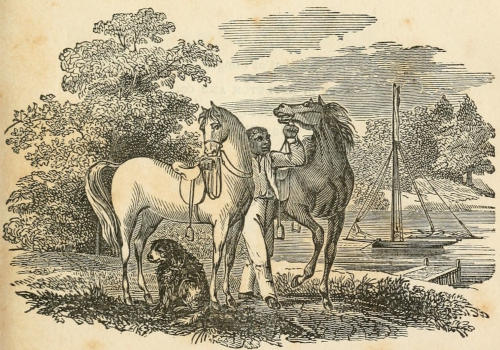This horizontally oriented, black-and-white drawing, possibly from the mid-1800s, features a central figure of a man, who appears to be of African descent, holding the bridles of two horses—one lighter and one darker—on either side of him. Both horses are saddled, suggesting they are ready for riding. Underneath the lighter horse sits a shaggy, dark-colored dog. The ground beneath them is depicted with detailed lines and shadowing, filled with foliage and shrubbery. In the background, a small sailboat is anchored on a calm body of water, with a pier extending out to the right of the darker horse. The scene is framed by large trees on the left and smaller trees on the right, beneath a sky dotted with clouds. The artwork is rendered on a light cream or tan-ish background, using a technique that employs vertical, horizontal, and diagonal lines to create detailed shading and texture.